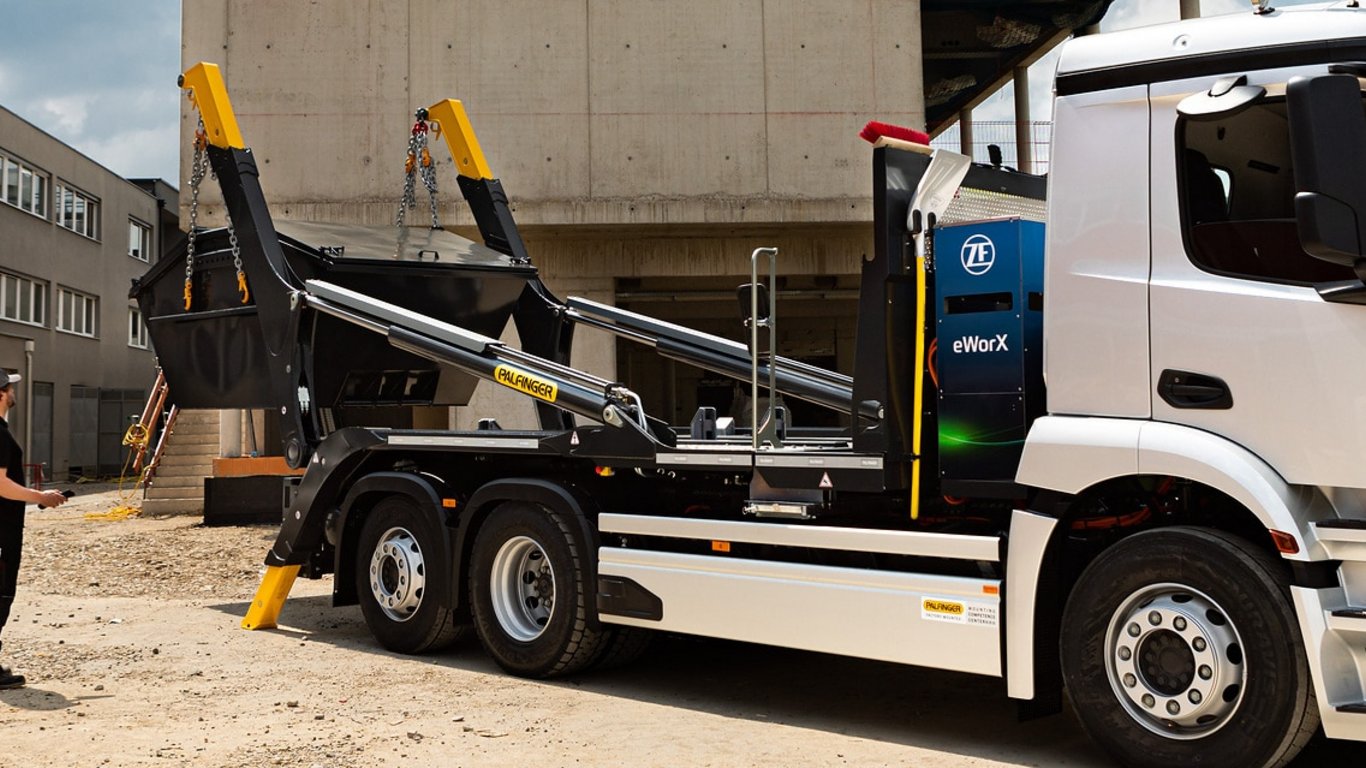This photograph features a large white truck with a distinctive cab and a flatbed designed for heavy hauling. The truck's right side displays three visible wheels, indicating its robust construction. Prominently, at the back of the truck, there are two hydraulic arms equipped with chains, which are connected to a large, shiny black metallic container. The container, which has angled flap doors on top, resembles a casket or small dumpster but is more refined and flatter in shape. The hydraulic arms are mainly black, with some parts painted yellow, and are crucial for lifting and securing the container. A man dressed in black, wearing a black hat, stands nearby, closely observing the operations. The ground beneath the truck shows slight disturbances, but no significant digging, implying a minimal impact on the surface. The truck's brand, PALFINGER, is visible, reflecting its suitability for such heavy-duty tasks.